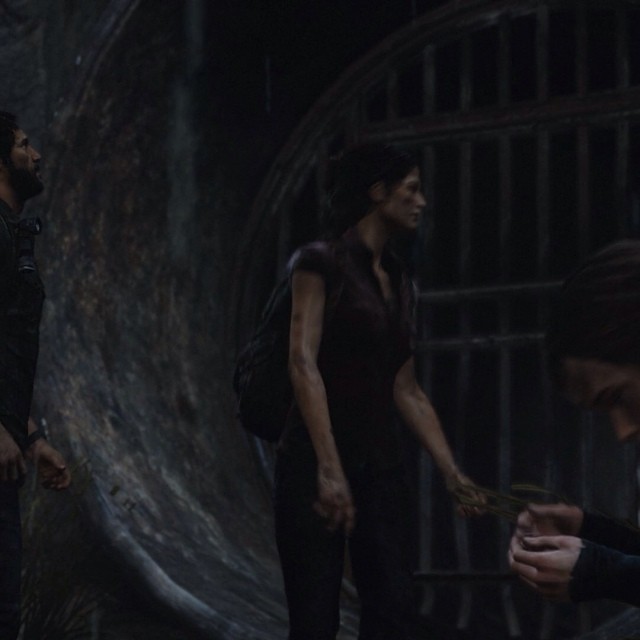This image is a computer-generated scene, likely from the video game "The Last of Us." It depicts three characters in a detailed 3D environment resembling a sewer area with metal bars and a circular structure in the background. In the center stands a female character wearing a red shirt, black pants, and a backpack. She has brown hair pulled back in a low ponytail and is possibly about to sacrifice herself to help the others. To the left, a male character with a beard and a black jacket gazes upward, wearing a watch. On the right, only the hands and upper face of another character, showing his eyes and a bit of his hair, can be seen. The setting adds tension, suggesting an imminent threat or critical moment in the narrative.